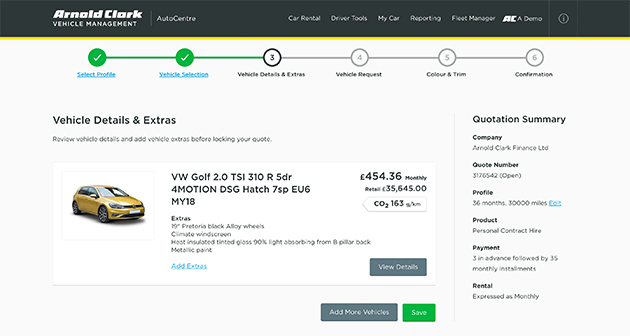This screenshot captures the Arnold Clark Auto Center Vehicle Management page, specifically highlighting various functionalities available for managing vehicles. The top menu features a sleek black bar with white text, presenting several clickable options that run left to right: "Car Rental," "Driver Tools," "My Car," "Reporting," "Fleet Manager," followed by the Arnold Clark logo abbreviated as "AC," and the word "Demo."

Below the main menu, the page displays a navigation process for managing vehicles. A specific profile has already been selected, indicated by a blue "Select Profile" link. The process is currently at the "Vehicle Selection" stage, the second phase. Beneath this, there is a prominent image of a vehicle accompanied by a heading labeled "Vehicle Details and Extras," providing more specific information and additional options related to the selected vehicle.